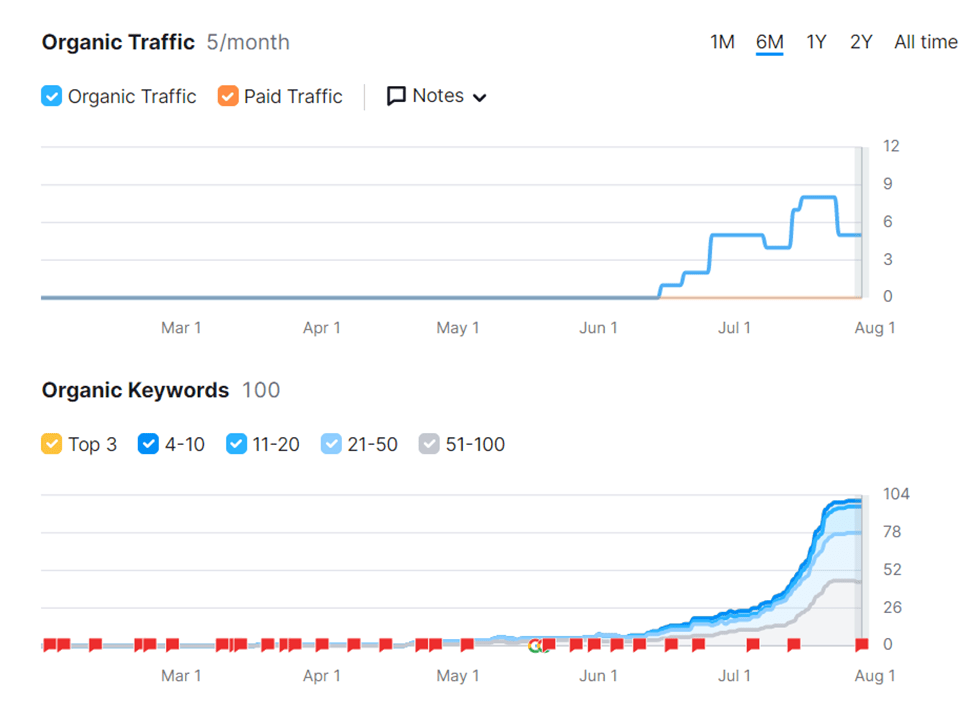This image depicts two line graphs stacked vertically. The upper line graph is titled "Organic Traffic (5 Months)" and displays data points corresponding to monthly organic traffic over a six-month period, with toggle options for time frames ranging from one month to all time. The "6 months" option is currently selected, indicated by a blue underline. The data starts at zero from March 1st through April 1st and May 1st, before increasing gradually mid-June: it ascends stepwise from zero to one, then to two, before jumping to five around July 1st. A slight decline to four occurs mid-July, followed by a sharp rise to eight, and finally dropping back to five by August 1st.

The lower graph, labeled "Organic Keywords (100)," shows a somewhat similar pattern. Starting around June 1st, the lines exhibit a steady, gradual increase, maintaining this upward trend until August 1st. The graphs collectively illustrate the organic traffic and keyword trends over the specified period, reflecting fluctuations and notable changes in data.